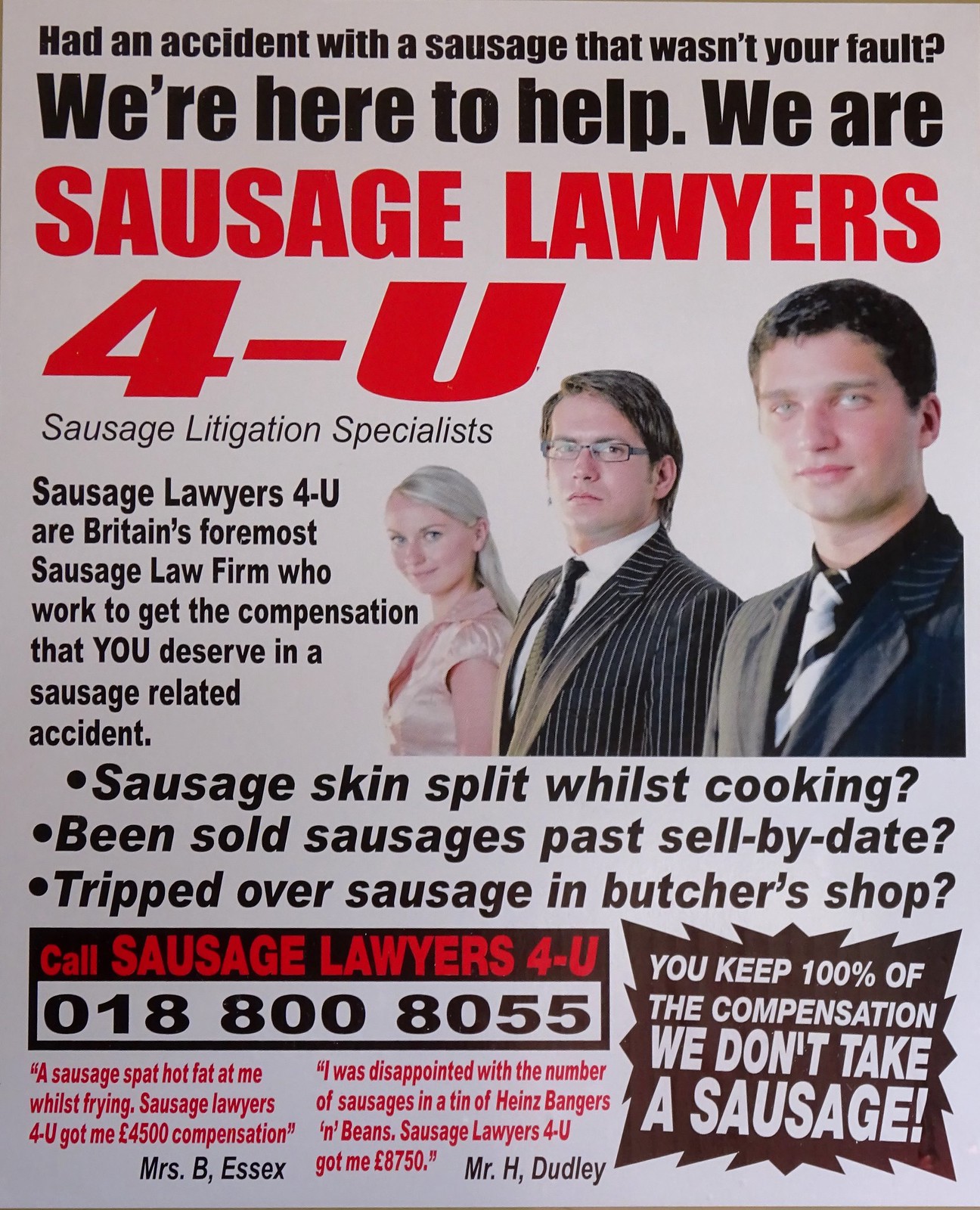This image portrays a whimsical advertisement that seems to parody legal services, specifically targeting humorous "sausage-related" grievances. The flyer is predominately whitish-gray with eye-catching red and black print. At the top, bold black text asks, "Had an accident with a sausage that wasn’t your fault?" followed by a reassuring message, "We’re here to help," in bold print.

The headline screams, "SAUSAGE LAWYERS 4-U," in large, bold red letters, followed by the tagline, "Sausage litigation specialists." The text brags that they are "Britain’s foremost sausage law firm" dedicated to securing compensation for various sausage mishaps. Examples include "Sausage skin split while cooking," "Been sold sausages past sell-by date," and "Tripped over a sausage in a butcher shop." Testimonials add humor, such as a case where "Sausage Lawyers for you got me £4,500 compensation. — Mrs. B. Essex." 

To the right of the text stand three attorneys: a woman, a man in a striped suit, and a man in a dark black suit. The man in the middle displays a serious demeanor, contrasting with the two at the ends who appear to be laughing. The overall playful tone is emphasized by the tagline at the bottom, "You keep 100% of the compensation. We don’t take a sausage," presented in white text within a black box.

The flyer’s layout uses varied font sizes and colors for emphasis, adding to its dramatic and humorous flair.